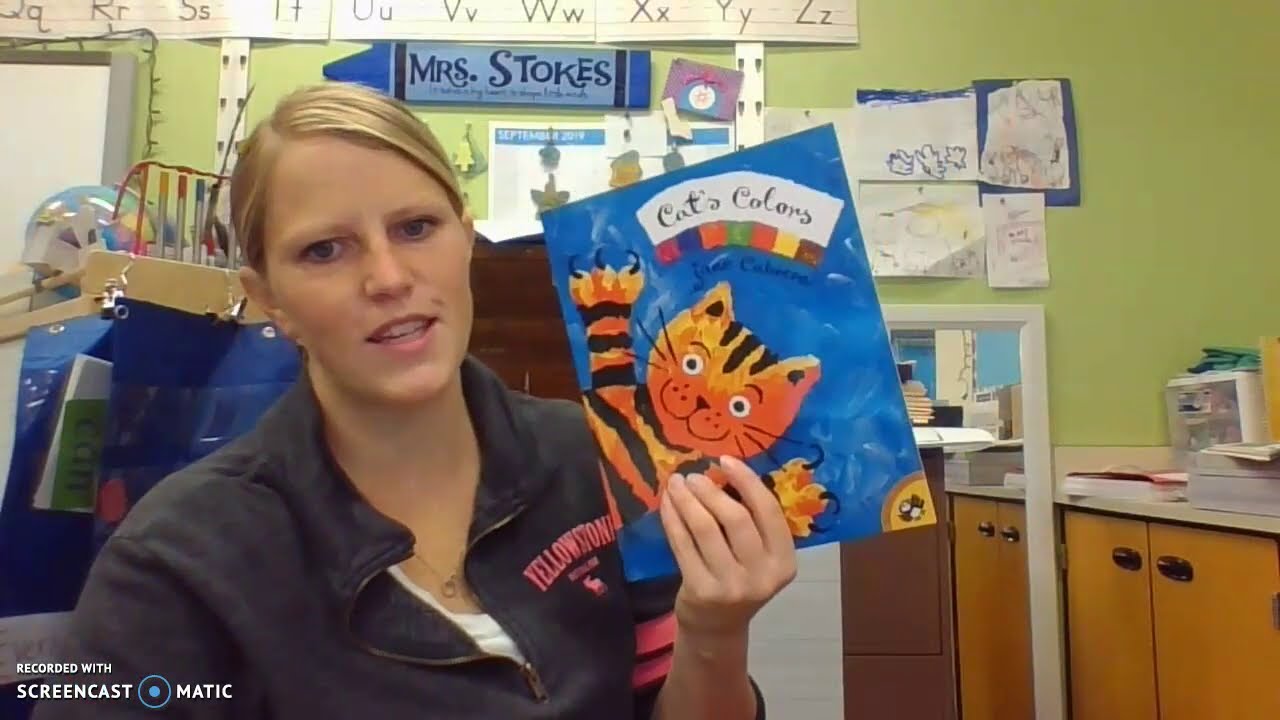In the image, a young woman, presumably a teacher named Mrs. Stokes, is conducting an online class, as indicated by the white text in the lower left corner reading "Recorded with Screencast-O-Matic." She has blonde hair tied in a ponytail and is wearing a gray jacket with the word "Yellowstone" in pink letters on the left breast, over a white shirt. She holds up a book with her left hand, titled "Cat's Colors," featuring an orange cat with black stripes set against a blue background. The cat on the cover has a smiling face with its arms extended. Mrs. Stokes is sitting in a classroom filled with colorful decorations, including numerous children's drawings pinned to a green wall behind her. There's a whiteboard to her upper left and a set of cabinets and a counter with various objects, such as a printer, to her right. A set of alphabet letters is displayed at the top of the wall.